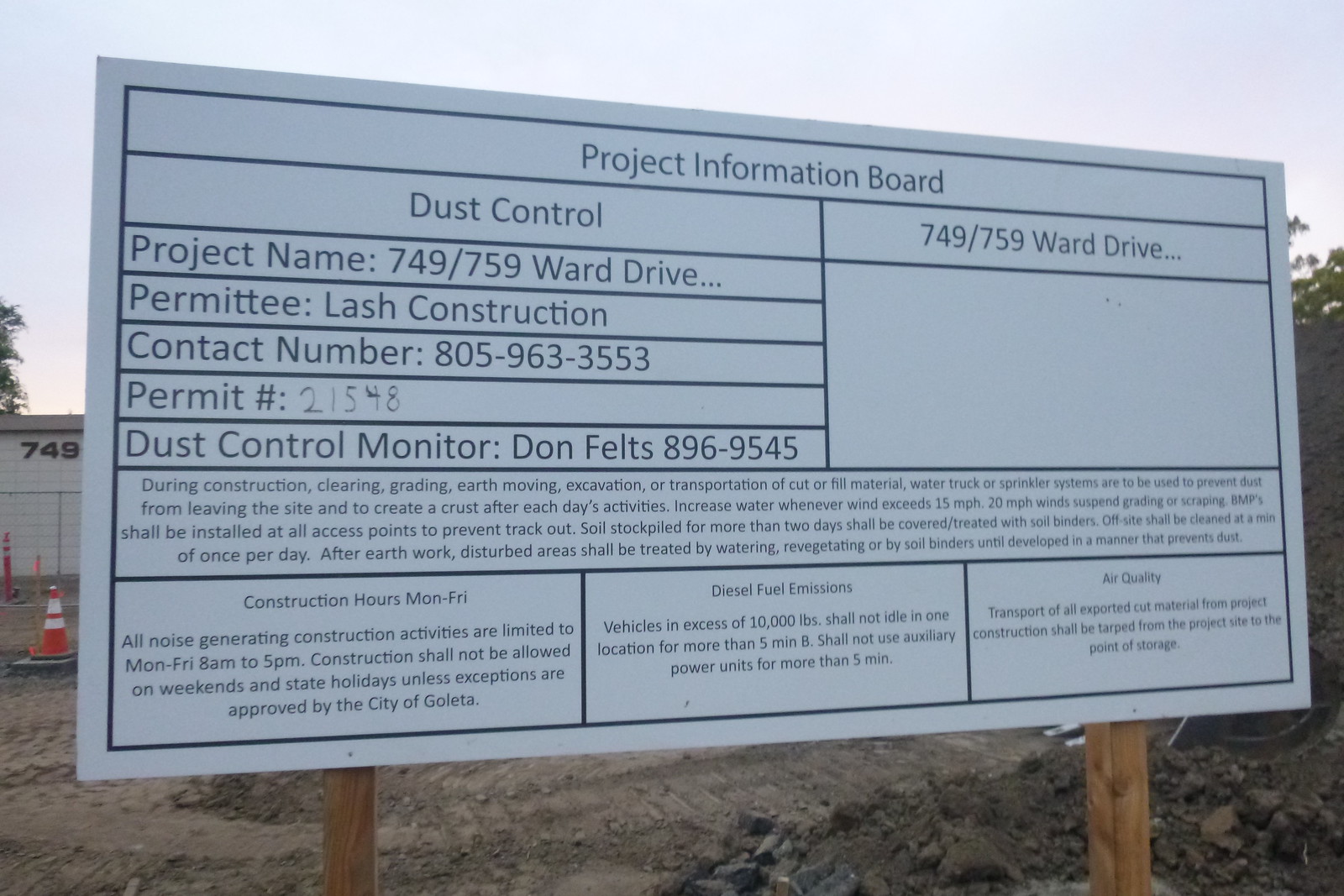The photograph features a large white billboard with a distinct black grid, displaying various pieces of information relevant to a construction site. Prominently titled "Project Information Board," it stands supported by two wooden posts. On the left-hand side at the top, the information grid starts with "Dust Control," and directly below is a series of squares containing specific details about the project. 

Details listed include the project name, permittee which is LASH Construction, contact phone number (805-696-3355), permit number (21548), and Dust Control Monitor Don Feltz along with his contact information. Further down, there's extensive text providing additional project information, including operational details such as construction hours, which are Monday through Friday from 8 a.m. to 5 p.m., with noise-generating activities restricted to these times. It explicitly states that construction is not allowed on weekends or holidays. Additionally, it notes that vehicles over 10,000 pounds are prohibited from idling at the site for more than 5 minutes.

On the right-hand side of the billboard, it displays the address, "749 to 759 Ward Drive." The sign stands against a backdrop featuring a large disturbed earth area, enclosed by a chain-link fence with visible cones marking the perimeter.